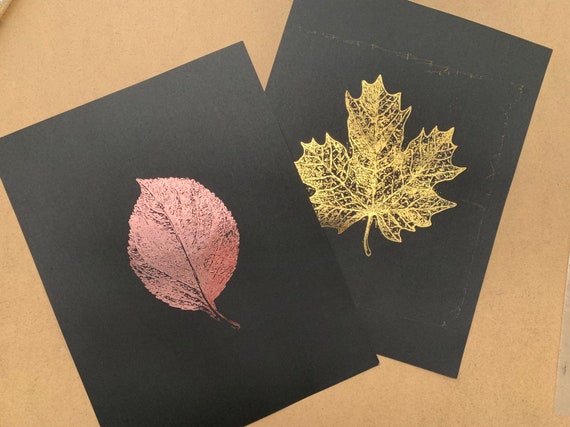In this photograph, a brown square background showcases two pieces of black cardstock, intricately adorned with foil-stamped leaf designs. Positioned diagonally on the left side is a piece of black cardstock featuring a meticulously detailed gold foil maple leaf, capturing the distinct veining. Slightly overlapping this and tilted to the left, the second piece of black cardstock displays a rose gold foil leaf. Both leaves, with their reflective, shiny textures, stand out prominently against their black backdrops, creating a visually striking contrast on the beige surface, which resembles the top of a table.